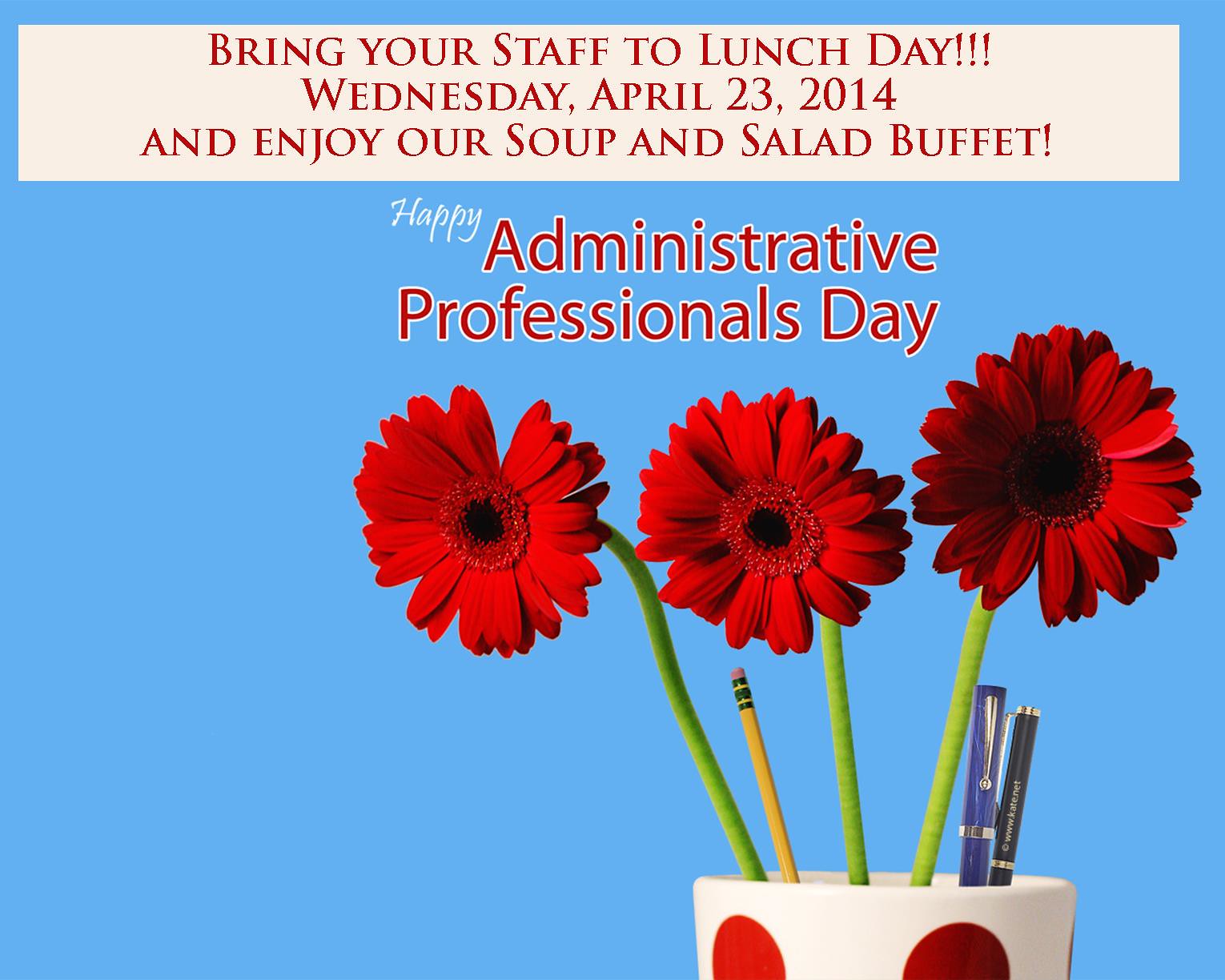The image features an advertisement likely from a magazine or website, set against a light blue background. Dominating the top 20% of the image is a white-striped banner with bold red lettering that reads, "Bring Your Staff to Lunch Day," and specifies the date as Wednesday, April 23rd, 2014. Below the banner, the ad encourages readers to "Enjoy our Soup and Salad Buffet" in the same red font.

Beneath this, on the light blue background, the message "Happy Administrative Professionals Day" is displayed in a lighter red text just above a central arrangement. At the center of the image, a white cup with red dots—holding two pens (one blue and one black) and a pencil—serves as a pen holder. Three artificial red flowers with green stems are also set in the cup, adding a pop of color and complementing the red lettering of the text.